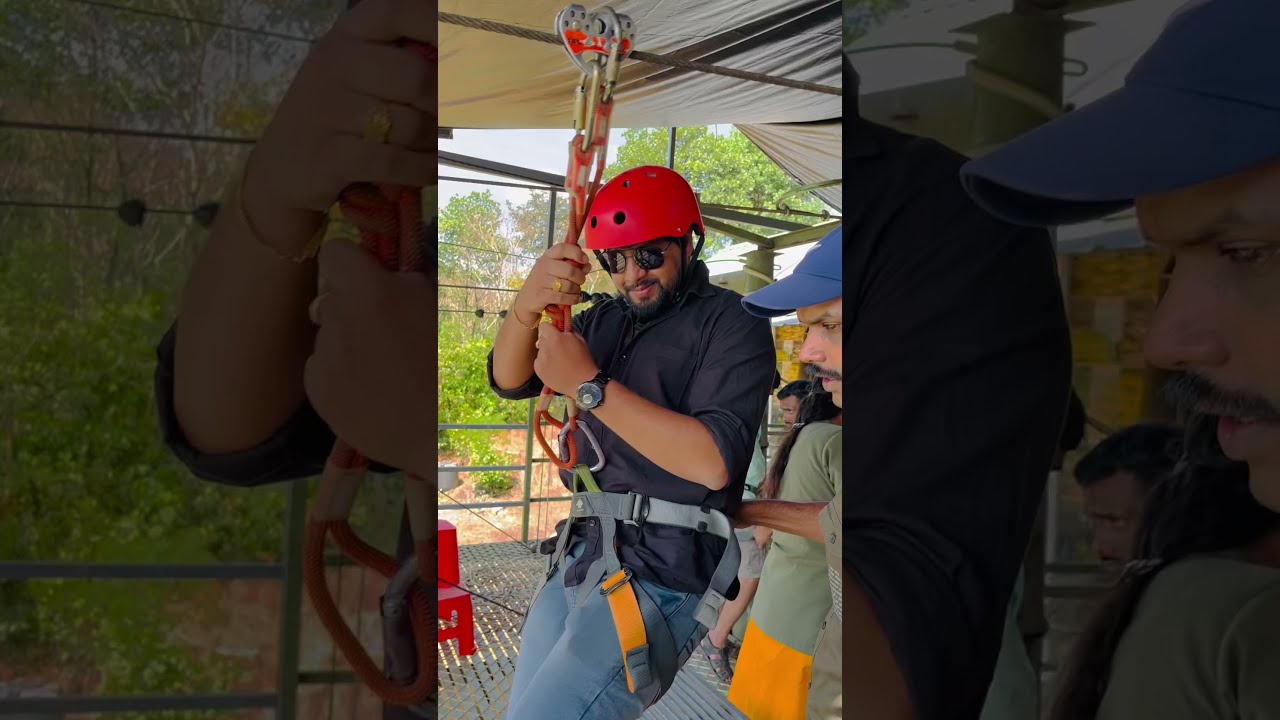The image is vertically oriented and divided into three sections, with the first and third showing darkened close-ups of the central section. In the middle is a detailed photograph of a man preparing for a zip line adventure. He is wearing a red helmet and shiny black sunglasses that cover his eyes above his dark beard. His olive-toned skin contrasts with his dark, likely navy, long-sleeved button-down shirt, which he has rolled up. The man is clad in safety gear, including a gray belt harness and safety straps that attach to a large carabiner and are connected to a zip line cable above him. He has grayish-blue pants and a wristwatch, and he clings to the harness with a slight smile on his face. Positioned on a metal platform under a canopy or tent, the scene includes another man to his right, sporting a blue baseball cap and a mustache, possibly an attendant. In the background, bright sunlight filters through green trees, adding to the adventurous atmosphere of the scene.